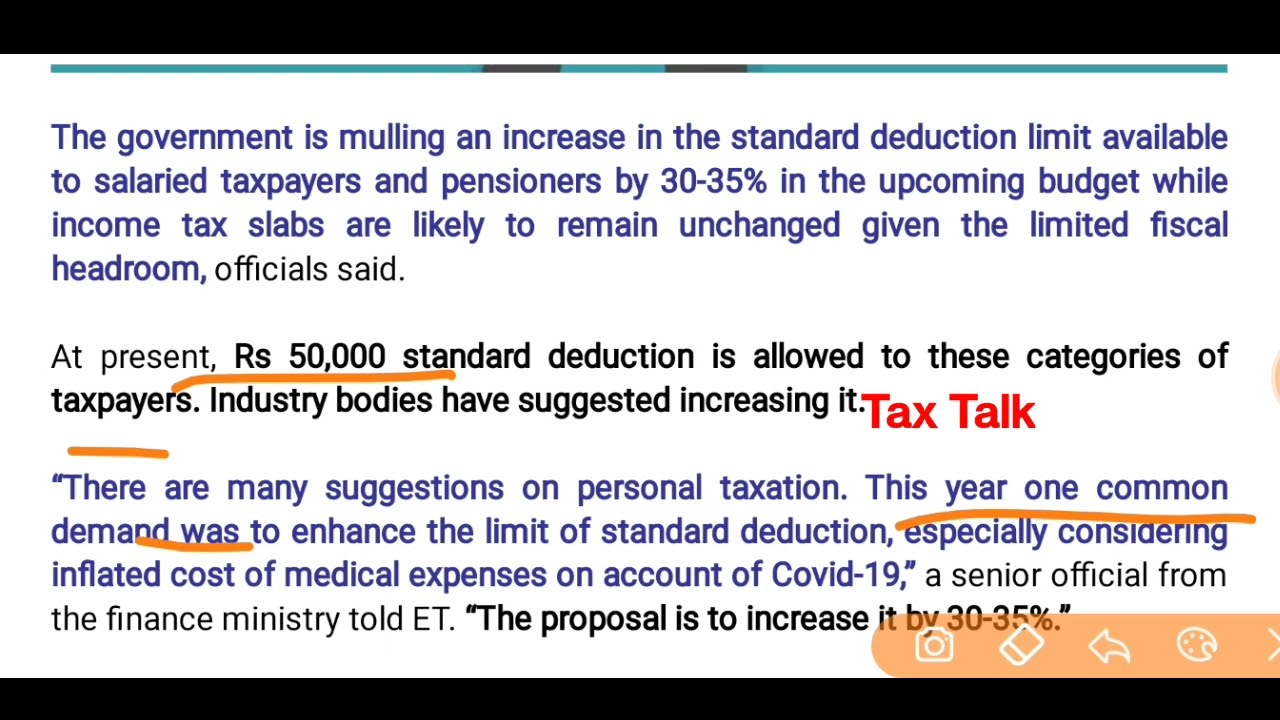The image is a white rectangular shape with a black stripe across the top and bottom edges. Inside the rectangle, there are three rows of text. The first paragraph is written in blue, stating that the government is considering increasing the standard deduction limit for salaried taxpayers and pensioners by 30 to 35% in the upcoming budget, while income tax slabs are likely to remain unchanged due to limited fiscal headroom, according to officials. The second paragraph, in black text, mentions that currently, a standard deduction of Rs 50,000 is allowed for these taxpayers, and industry bodies have suggested increasing this amount. The third paragraph, in blue with some black text, includes quotes from a senior official from the finance ministry, noting that there have been many suggestions regarding personal taxation this year, with a common demand being to enhance the standard deduction limit, especially considering the increased medical expenses due to COVID-19. It concludes with a proposal to increase this limit by 30 to 35%. Various parts of the text are underlined in red, and the lower right-hand corner features an orange stripe containing white icons of a camera, an arrow, and a paint palette.